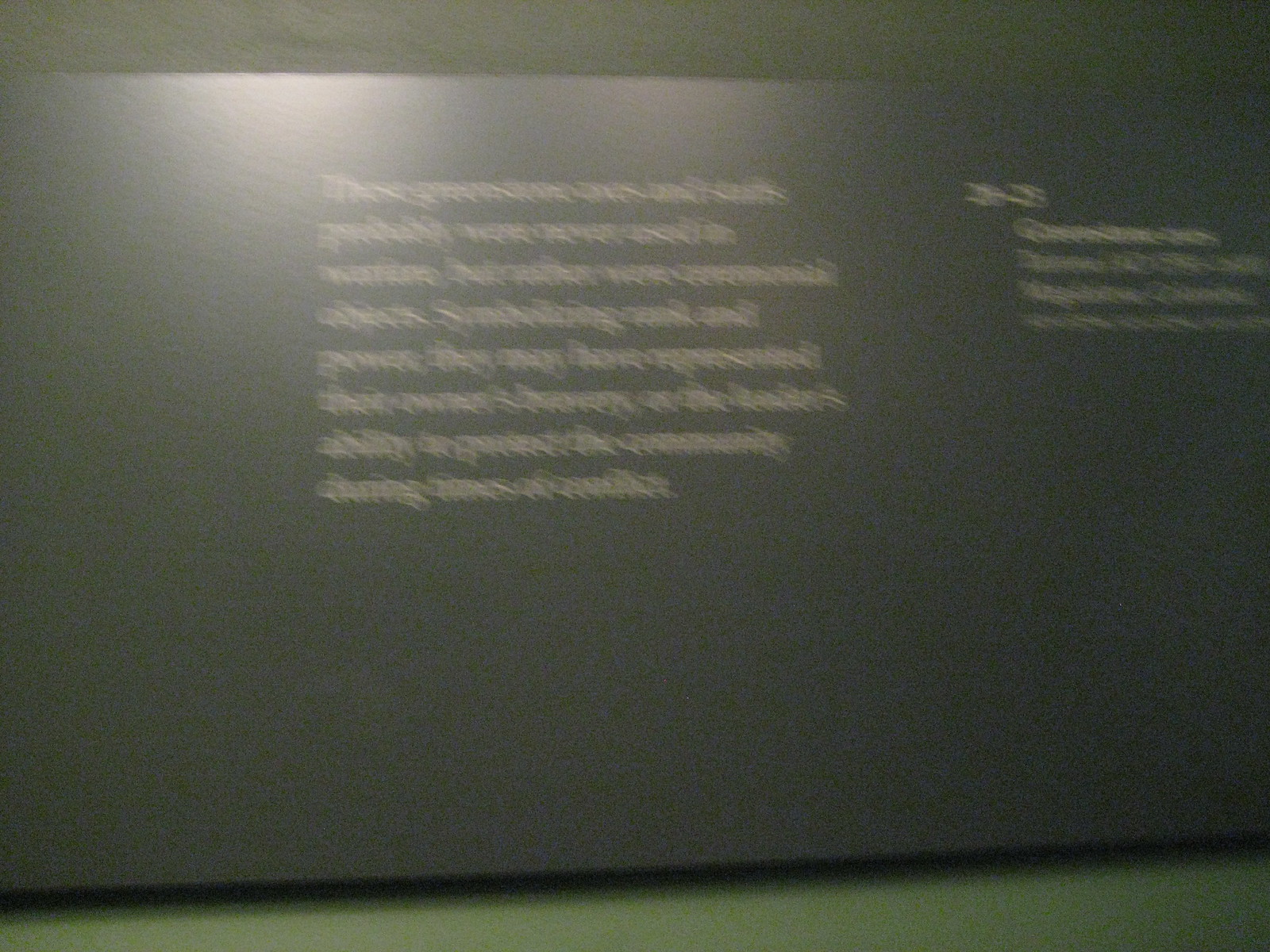This rectangular image captures a photograph of an engraved inscription on what appears to be a stone or marble wall. The engraving, rendered in a dark olive green hue, features nine lines of text that run vertically from top to bottom. Although the text is illegible due to the blurriness of the image, it seems to be a series of phrases or names. To the right of this main inscription, there are an additional four lines of text in a lighter green color, equally unreadable because of the blurriness.

At the bottom of the photograph, a thin strip of lighter green, possibly also stone or marble, is visible. The top portion of the photograph is framed by a darker shade of green. Natural light illuminates the top third of the image, adding contrast to the overall scene.